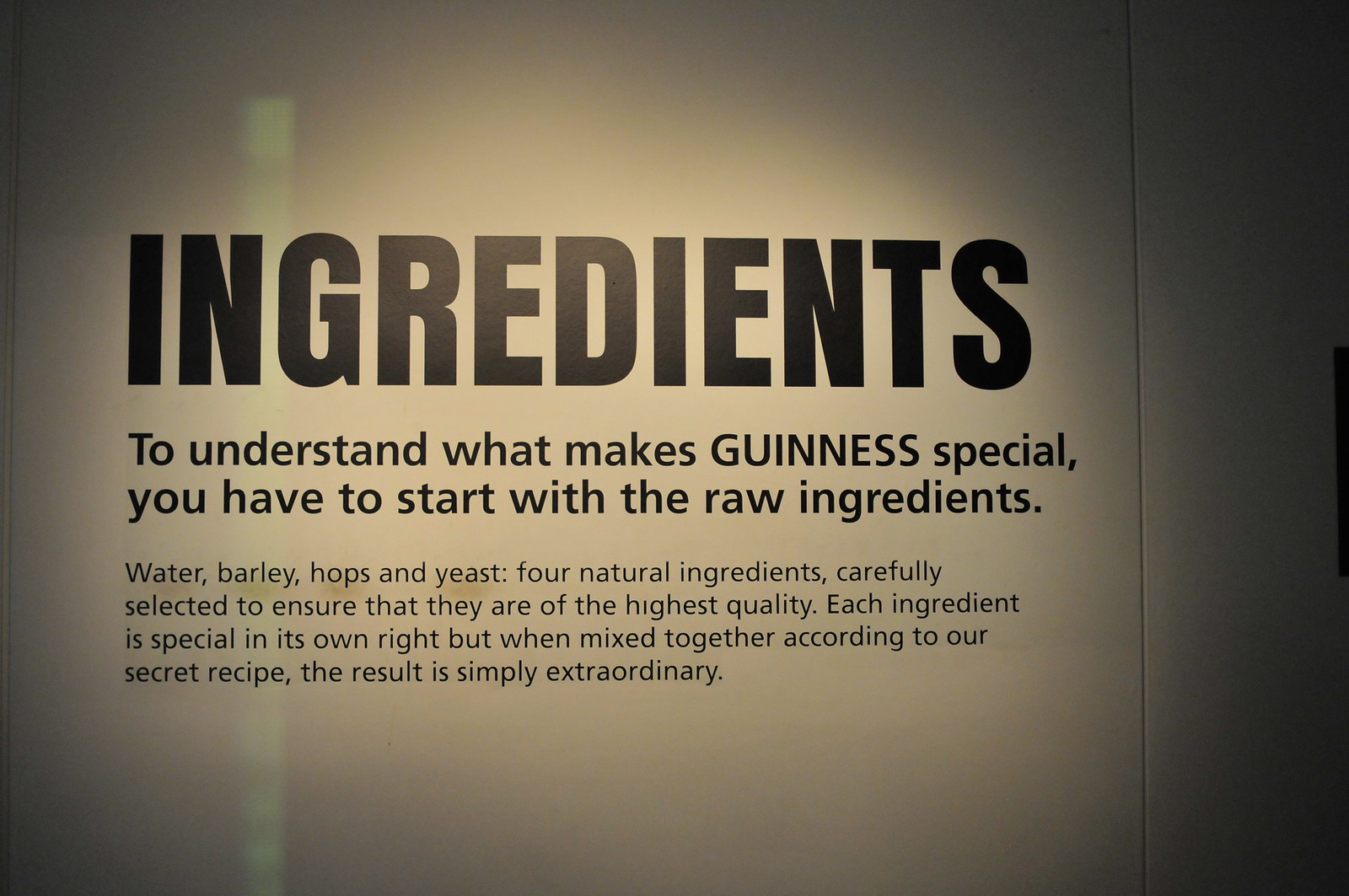The image features a close-up of a text-based display, reminiscent of a museum exhibit, against a tan or off-cream background with shadows and glares suggesting it is photographed through glass. Bold black font at the top prominently reads "Ingredients." Below it, in slightly smaller black font, it continues, "To Understand What Makes Guinness Special, You Have to Start With the Raw Ingredients." Further down, in even smaller black text, the description reads: "Water, Barley, Hops, and Yeast. Four Natural Ingredients, Carefully Selected to Ensure They Are of the Highest Quality. Each Ingredient is Special in Its Own Right, but When Mixed Together According to Our Secret Recipe, the Result is Simply Extraordinary." A green glare streak runs from the top to the bottom of the left-center side, enhancing the impression of viewing a refined presentation through a glass surface.